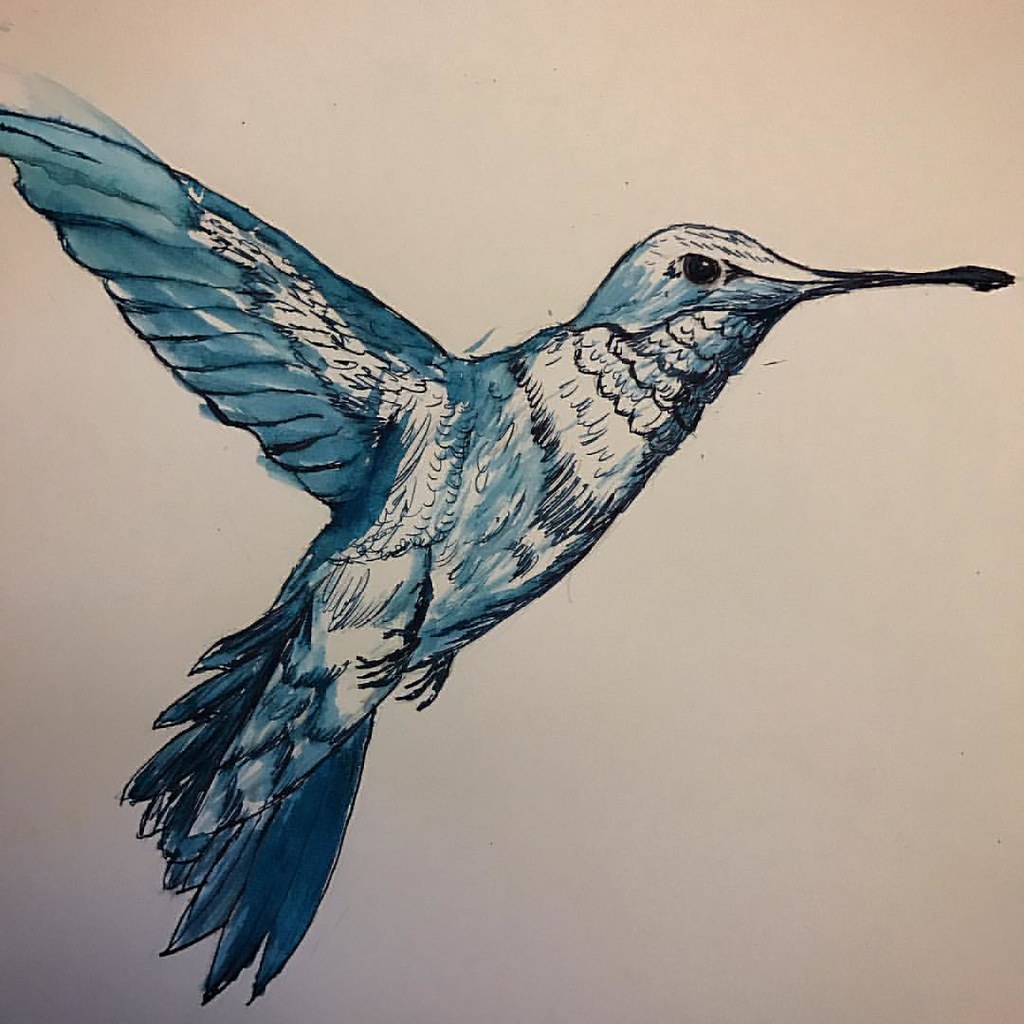This is a detailed, color photograph capturing a meticulously inked line drawing of a bird. The bird is depicted facing the right, with a very long and thin beak, and its eye is distinctly visible. The artist has intricately illustrated multiple layers of feathers on the bird's breast and wings. The feathers have been selectively colored using various shades of dark, steely blue and black, giving the bird a striking, albeit partially colored, appearance. 

The background color is difficult to ascertain due to the artificial lighting in which the photograph was taken, causing it to appear darker than it likely is. In the lower left corner of the image, the background transitions to an almost dark grey hue, though it is probable that the original medium could be white or grey paper.

Additionally, there is a subtle blue mark where the wing meets the bird's back, suggesting a slight coloring error. A few minor pencil scratches are also present, notably one just under the bird's beak. Despite these small imperfections, the overall composition highlights the detailed and thoughtful approach taken to render this avian subject.